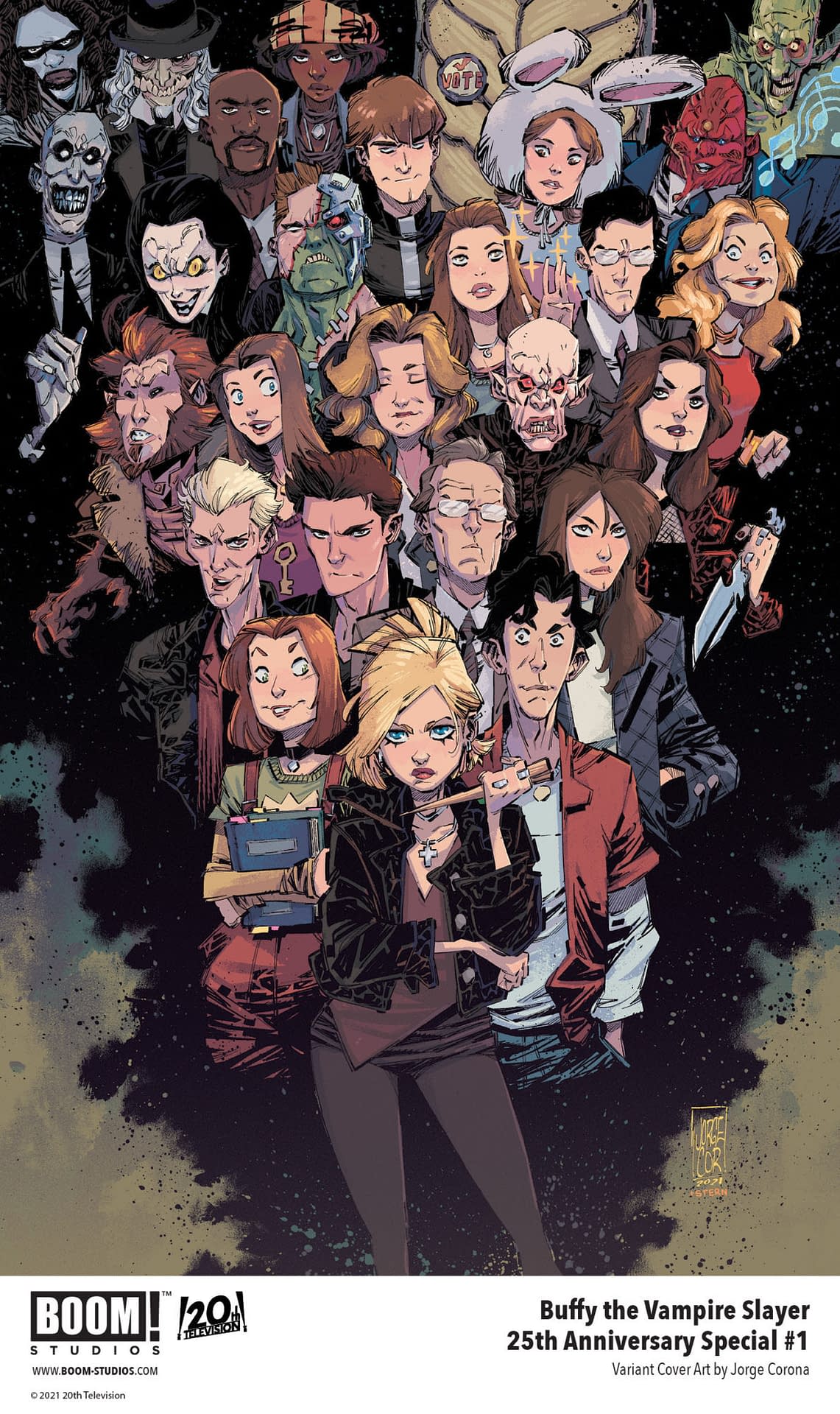The image is the variant cover for the "Buffy the Vampire Slayer 25th Anniversary Special Number 1," with artwork by Jorge Corona. Central to the composition is Buffy herself, identifiable by her blonde hair tied up, her black leather jacket, and the stake she is holding. The characters are arranged in a V-shaped formation with Buffy in the forefront. Notable characters include Willow in red overalls holding a book, Xander in a red shirt with a white shirt underneath, Angel, Spike, and various other figures from the series like a woman in a bunny suit, a human-robot hybrid, and ghouls, reflecting a diverse array of characters from the "Buffy the Vampire Slayer" universe. The bottom of the image features logos from Boom Studios and 20th Century Fox, with the copyright reading 2021, 20th Television.